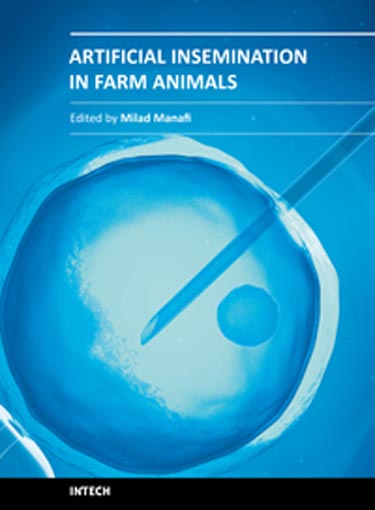The image displays an academic-style book cover for "Artificial Insemination in Farm Animals," edited by Milad Mahamfi. Dominated by tones of light blue, dark blue, and white, the cover features a detailed illustration of an egg cell being injected with an embryo via a hypodermic needle. The embryo, positioned on the left side, extends to nearly the right edge and over halfway up the image. At the center of the egg cell, a bright nucleus is visible. The title and editor's name are written in white sans serif font against the blue gradient background, with additional decorative lines around the text. A black banner at the bottom contains the publisher's name, "InTech," in white text. The overall impression suggests that the cover belongs to educational course material or a pamphlet focused on the artificial insemination of farm animals.